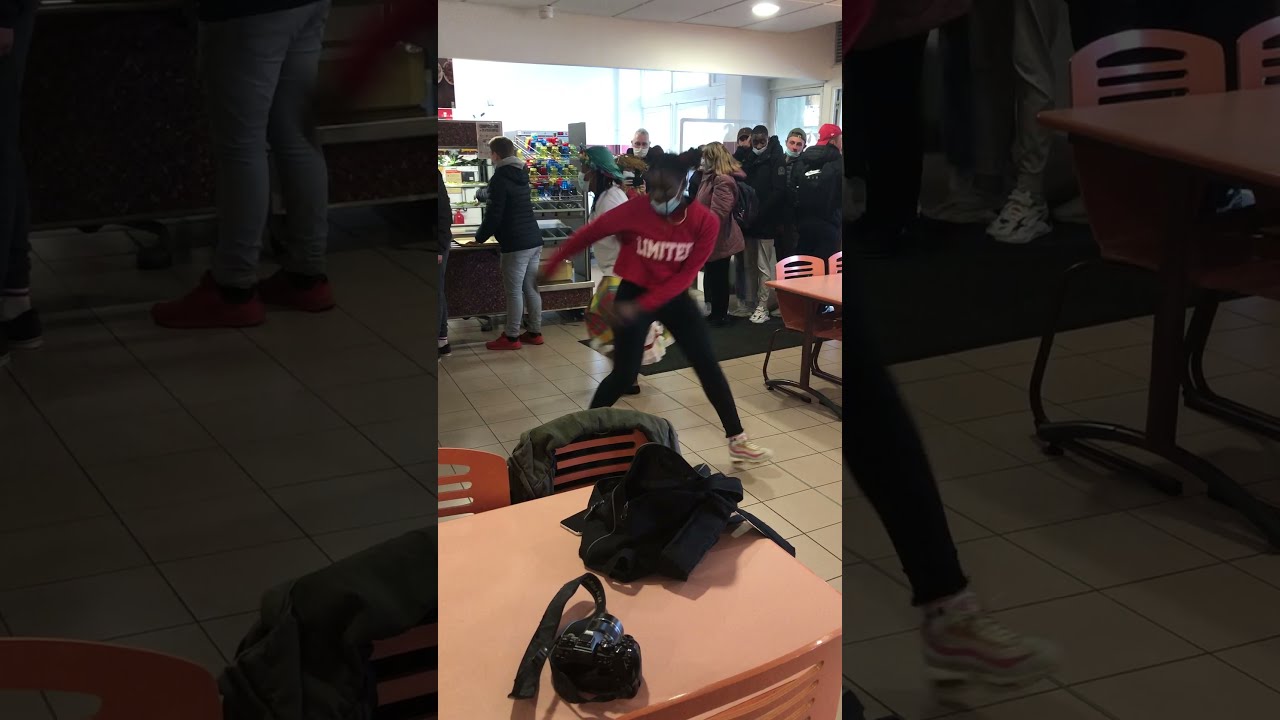The image depicts a lively scene inside what appears to be a middle or high school cafeteria. At the center of the photo is an African American girl, dancing. She is wearing a red, long sleeve shirt with white writing that seems to say "limits are limited" along with black leggings and a COVID mask. Surrounding her, several teenagers are standing in line, likely to pick up food. Most of them are also wearing masks and black jackets. In the foreground, there is a brown table with chairs, on which a black purse and a jacket are placed. The setting features a tan tile floor, additional tables and chairs, refrigerators with stored items at the back, and overhead lights that brighten the room. The color palette in the image includes shades of pink, black, brown, tan, gray, red, white, green, blue, and light blue. Notably, there is a dark-colored rug at the entrance of this indoor location, which is likely a bustling cafeteria.